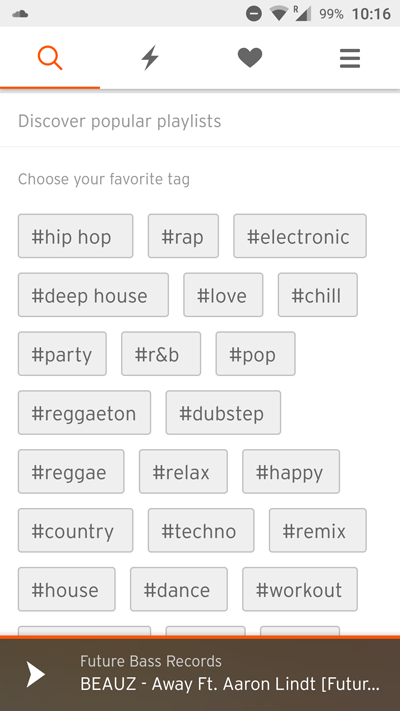### Detailed Descriptive Caption for Music Application Screenshot:

The screenshot captures the user interface of a music application on a smartphone. At the top of the screen, several icons are visible: a Google Cloud icon on the upper left, an unidentified icon featuring a circle with a bar through it, followed by a Wi-Fi signal beacon, a battery icon indicating 99% charge, and the current time displayed as 10:16. 

Below these indicators, there are four major navigation icons arranged horizontally. The leftmost icon, an orange magnifying glass with an orange bar underneath, is highlighted to indicate it is currently selected. The other icons depicted in grey are: a lightning bolt, a heart, and a hamburger menu. Beneath these icons, a thin grey line marks the start of the main content area.

The first section of the main content area contains the text "Discover Popular Results" in grey, followed by "Choose Your Favourite Tag." Below this, a variety of music tags are displayed within peach-colored button fields, each outlined with a thin grey line. The tags include:
- #hip-hop
- #rap
- #electronic
- #deep house
- #love
- #chill
- #party
- #R&B
- #pop
- #reggaeton
- #dubstep
- #reggae
- #relax
- #happy
- #country
- #techno
- #remix
- #house
- #dance
- #workout

There are several more tags that require scrolling to view.

At the bottom of the screen, a thin orange line overlays a brown field, which contains information about the current track. The displayed text reads "Future Based Records" along with a play button. Below that, it lists the song "Bose (BEAUZ) - Away featuring Aaron Lint & Future [incomplete text]."